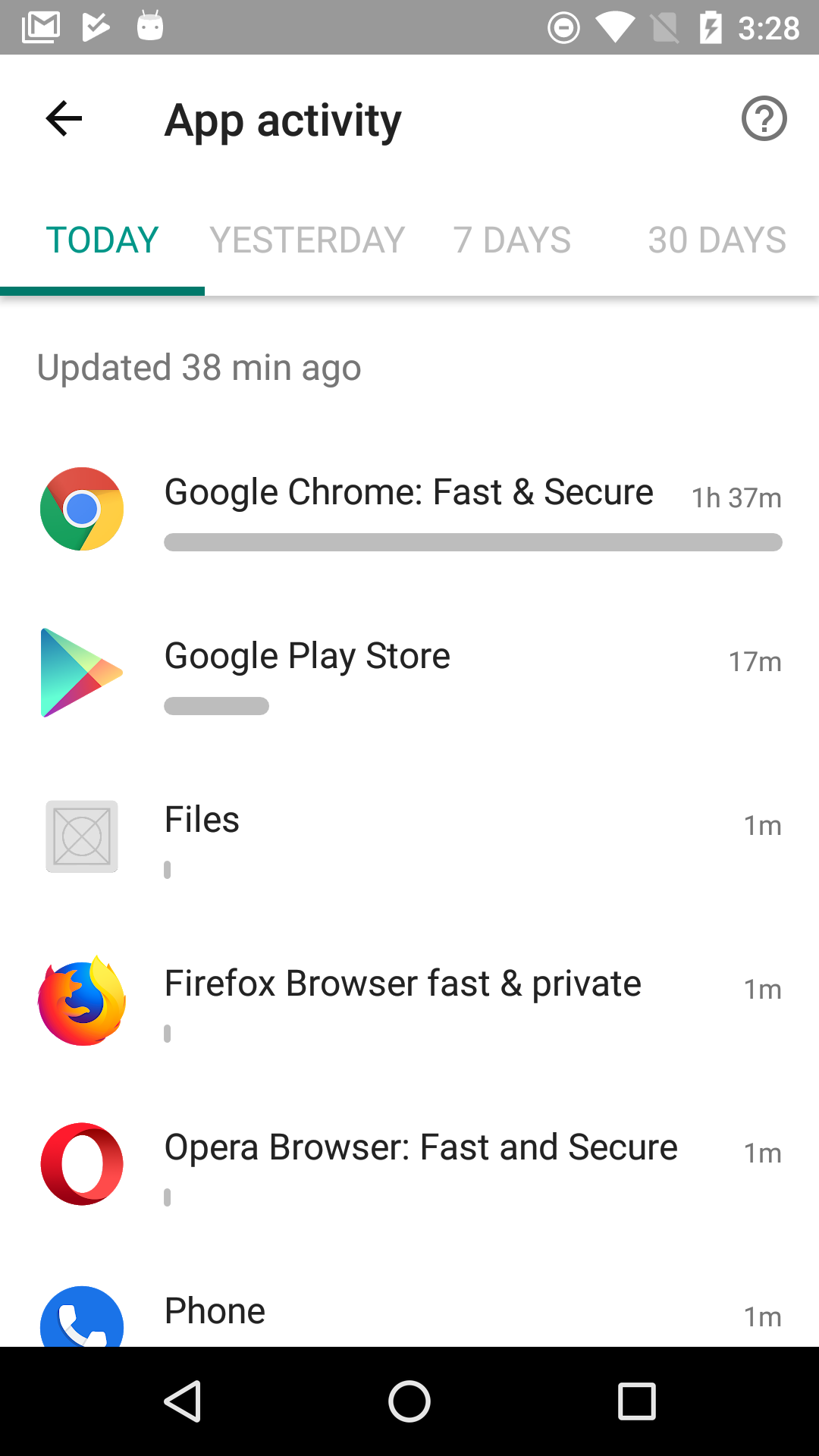The image is a detailed screenshot of a smartphone interface, capturing both the status bar at the top and a specific app activity summary. 

### Status Bar:
- **Left Side Icons:** Gmail, Play Store, and another icon resembling a bag with two dots inside it.
- **Right Side Icons:** Do Not Disturb, full Wi-Fi signal, a grayed-out SD card icon with a strikethrough, a vertical battery icon with a lightning bolt indicating charging, and the time displayed as 3:28 PM.
- **Color Scheme:** All icons and texts in the status bar are white on a gray background that spans the top portion.

### Main Screen:
- **Header Section:**
  - **Left:** A back arrow.
  - **Center:** The text "App Activity" in bold, black sentence-case letters.
  - **Right:** A dark gray question mark icon inside a circle.
- **Tab Menu:**
  - **Highlighted Tab:** "TODAY" in blue, capital letters with an underline.
  - **Other Tabs:** "Yesterday," "7 days," and "3 days" in light gray text, with a thinner gray line under the entire tab section.
- **Update Information:** "Updated 38 minutes ago” beneath the tab menu.
- **App Activity List:**
  1. **Google Chrome:** Icon in color, description "Google Chrome, fast and secure," usage time of 1 hour and 37 minutes, with a full progress bar.
  2. **Google Play Store:** Icon in color, usage time of 17 minutes, with a short progress bar equivalent to the width of the word "Google."
  3. **Files:** Icon resembling a square with an X inside a circle, usage time of 1 minute.
  4. **Firefox Browser:** Icon in color, description "Firefox Browser, fast and private," usage time of 1 minute.
  5. **Opera Browser:** Icon in color, description "Opera Browser, fast and secure," usage time of 1 minute.
  6. **Phone:** Blue circle icon with a white phone, usage time of 1 minute.

### Bottom Navigation Bar:
- Left to Right: Triangle (back), Circle (home), and Square (recent apps) icons, all set on a black background bar.

This detailed summary captures both the status and activity visible on the phone screen.